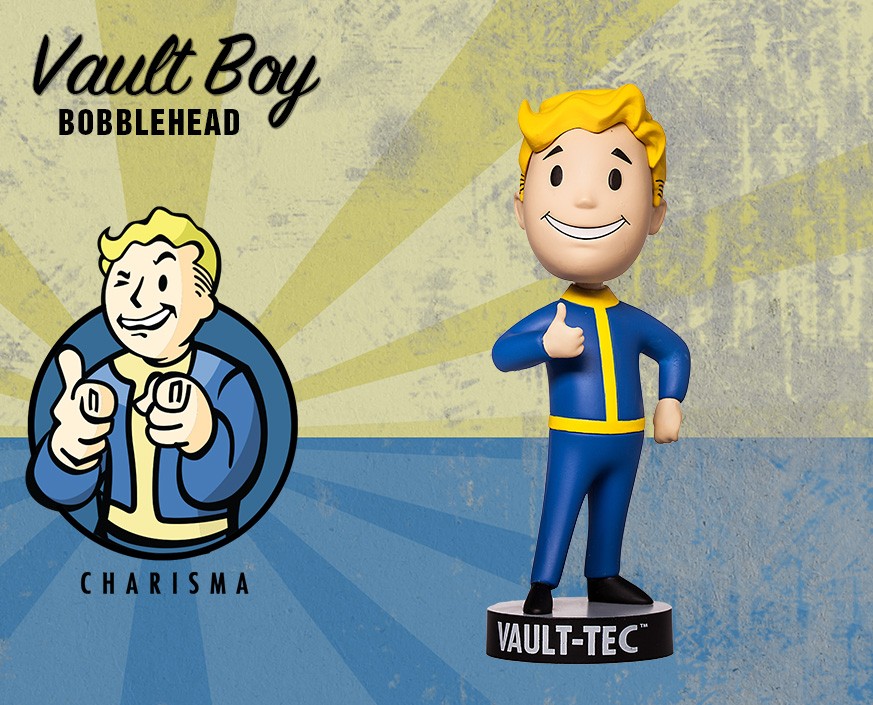This horizontal-rectangular image is a detailed illustration promoting a Vault Boy Bobblehead from the Fallout games. In the upper left corner, the text "Vault Boy" is written in cursive, with "Bobblehead" in block letters directly beneath it. Below this text is an in-game icon of Vault Boy characterized by his blonde hair, cheerful expression, and classic blue jumpsuit with yellow accents, giving a thumbs-up gesture. The word "Charisma" is capitalized in black letters underneath this image. On the right side, the bobblehead itself is depicted: the same boy with yellow hair, a big smile, wearing the blue and yellow outfit and standing on a pedestal labeled "Vault-Tec." The background features a faded paint design with a yellow upper half and blue lower half, reminiscent of an explosion or burst effect. The combination of these details creates a nostalgic and vibrant representation of the beloved Fallout character.